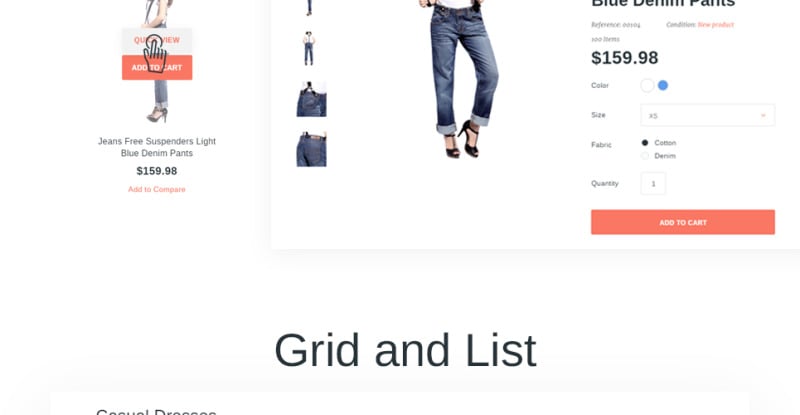Detailed Caption:

On the left side of the image, there is an "Add to Cart" button along with a detailed preview of light blue denim pants priced at $159.98. This preview includes a quick view button and a label indicating that free suspenders are included with the purchase. 

In the center, the main image displays a pair of blue denim pants, referred to simply as "Blue Denim Pants," also priced at $159.98. Directly below the main image, the color option of the jeans is prominently displayed, followed by the available sizes and fabric options, which include both cotton and denim. Below these details, there is a section to choose the quantity accompanied by an orange "Add to Cart" button. 

The jeans are showcased in blue, worn by a model complemented with black shoes. The product is provided with four different images, giving a comprehensive view of the jeans from various angles. The jeans are noted to be a new product, and a reference number is also provided.

Beneath this section, the background turns gray and includes words like "grid" and "list" at the bottom. The display is partially cut off, showing the text "casual dresses."